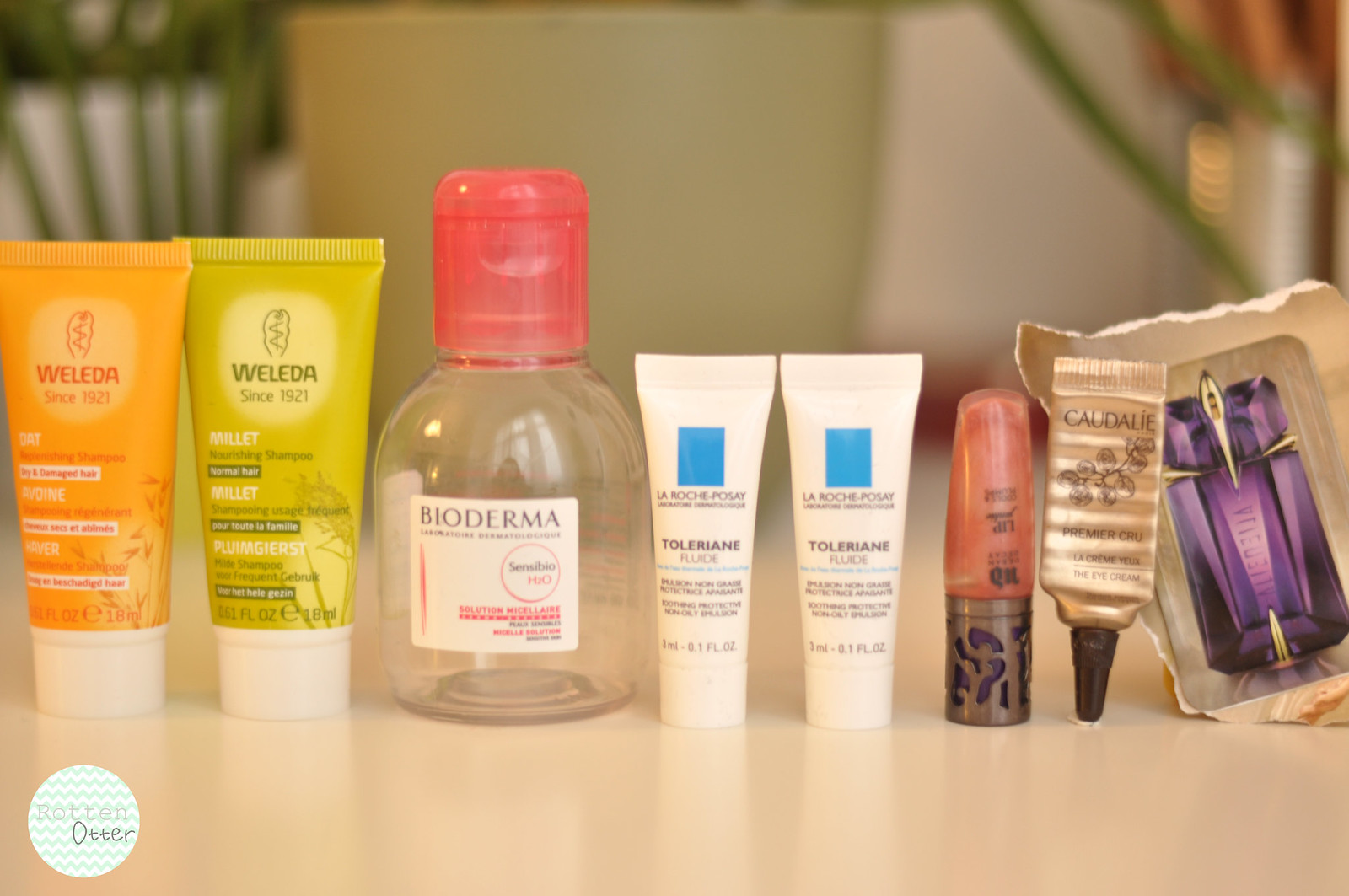The image showcases an array of beauty products meticulously arranged in a row on a cream-colored countertop. The warm, neutral tones of the counter make the products stand out. In the blurred background, there are hints of greenery and other indistinct items, adding a touch of calm and natural ambiance to the scene.

In the lower left-hand corner of the image, there is a small circular logo with a chevron pattern, featuring the words "Rotten Otter." This logo introduces the selection of products, adding a touch of personalized branding.

Moving from left to right, the first product displayed is Weleda Oat Replenishing Shampoo, packaged in a vibrant orange container with a twist-off cap. Next to it is another Weleda product, a Millet Nourishing Shampoo for normal hair, housed in a green bottle with a similar cap.

The third item is a bottle of Micellar Water by Bioderma. The container is clear, with a semi-transparent pink cap that brings to mind the translucent designs of 90s-era technology.

Following this, there are two La Roche-Posay Toleriane Fluid items. These are encased in small, white bottles adorned with a signature blue square above the brand name, though the precise wording is blurred.

Next, a lip gloss with a rose-patterned twist-off cap is barely discernible in the image. The exact branding is unreadable, adding an element of mystery.

To its right is a bottle of Caudalie Premier Cru Eye Cream. This product comes in a squeezable bottle with a precision twist-off tip, designed for targeted application.

The final item appears to be an irregularly cut picture with frayed edges, possibly torn from a magazine or product packaging. The image depicts a perfume bottle in a rich purple hue, adding an artistic and intriguing element to the collection.

This thoughtfully composed image captures a diverse selection of beauty products, hinting at both their functionality and the aesthetic sensibilities of their owner.